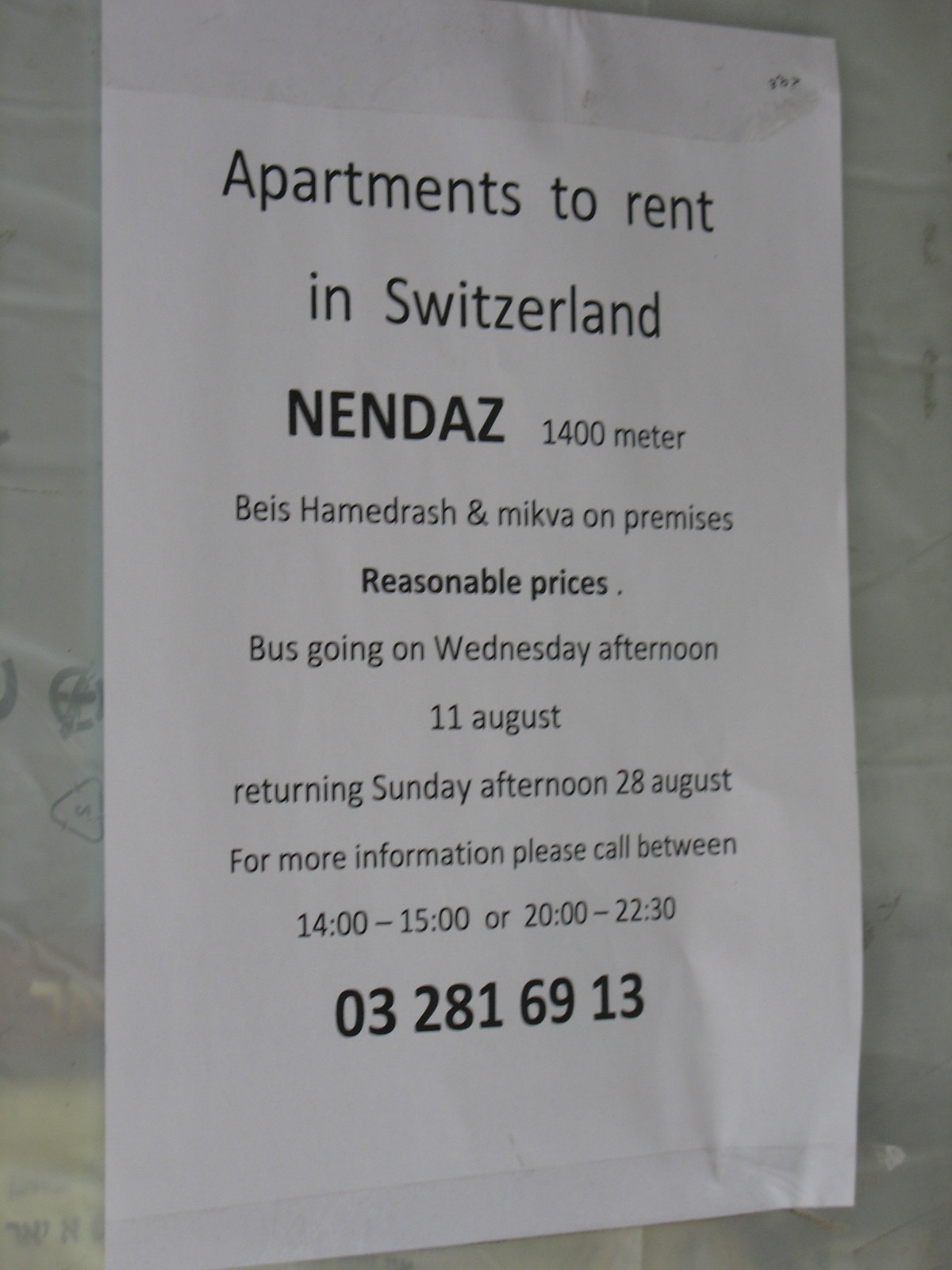The image displays a white piece of paper taped up to a white wall in what appears to be a lobby or student union. The notice is in black print and centers its text on the page. At the top, it reads "Apartments to Rent in Switzerland" with "NENDAZ, 1,400 meter" prominently highlighted in bold. Below that, it mentions "Beis Hamedrosh and Mikva on-premises" followed by "Reasonable Prices" also in bold. The notice further details that there is a bus going on Wednesday afternoon, 11 August, and returning Sunday afternoon, 28 August. For more information, it instructs readers to call between 1400-1500 or 2000-2230, providing a contact number: 032-816-913.